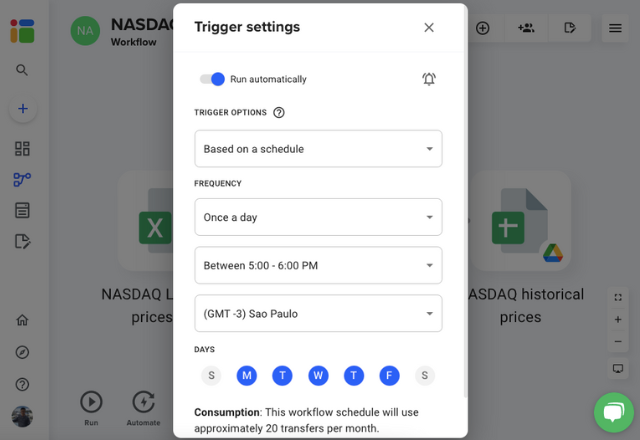The image shows an application launching on what appears to be a tablet, suggested by the nearly 4:3 aspect ratio typical of an iPad. The interface features a primarily white color palette set against a subtly grayed-out background, creating a floating effect for the central pop-up menu. This application identifies as the NASDAQ Workflow Application, and it displays various documents, including NASDAQ Historical Prices and other partially visible NASDAQ price documents.

On the left side of the screen, there is a grid of menu icons, while the top section contains another grid of icons, including a notable three-bar menu icon. The focal point, a pop-up menu titled "Trigger Settings," features a blue toggle switch labeled "Run Automatically," which is currently activated. Below this, the menu displays multiple configuration options under "Trigger Options," allowing the user to select "Based on a Schedule." The schedule options include:

- Frequency: Once a Day
- Time Range: Between 5:00 PM and 6:00 PM
- Time Zone: GMT-3 (Sao Paulo)

Further customization is available under "Days," where users can select specific days of the week to run the workflow. The selected days are Monday through Friday, highlighted in blue, while Saturday and Sunday are grayed out and not selected. At the bottom, a note under "Consumption" indicates that the current workflow schedule will use approximately 20 transfers per month.